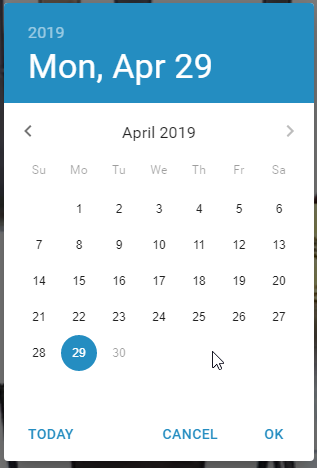The image depicts a screenshot with a vertically-oriented rectangle that has a slim dark gray border. At the top, there is a blue header featuring bold white text that reads "MUN for Monday, April 29th." Above the header, in small, very light blue text, the year "2019" is displayed. Below the blue header lies a white background featuring gray text that presents a calendar for the month of April.

In the center of the calendar, in bold, it states "April 2019," flanked by navigational arrows pointing left and right to browse to previous and next months. The calendar grid outlines all 30 days of April, with the 29th prominently highlighted in a blue circle.

At the bottom of the calendar, in blue text, the label "Today" sits on the left, indicating the current date. To the right, the options "Cancel" and "OK" are located at the lower right corner, allowing for interaction with the calendar.